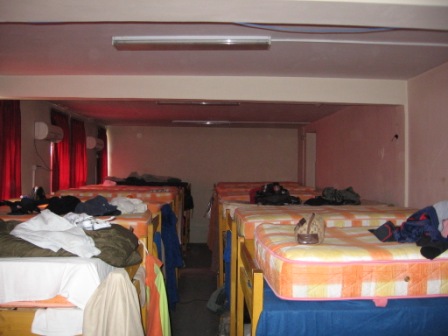This detailed caption provides a comprehensive description of the image:

The image depicts a cramped dormitory room with a very low ceiling, illuminated by limited light coming through drawn red curtains. The interior features two rows of bunk beds arranged in parallel, with approximately three to four beds in each row. Each bunk bed comprises two levels: the top mattress is covered with vibrant orange, yellow, and white plaid sheets, while the bottom mattress is draped with a blue bed skirt. The beds are cluttered with crumpled clothes and personal items, indicating occupancy. To the left side of the room are windows adorned with red curtains, and to the right, a stark pink wall. The backdrop includes a white wall, contributing to the enclosed, small-room atmosphere. The photograph captures the scene from an angle that faces directly at the rows of beds, framing the tight, busy environment of the dormitory.